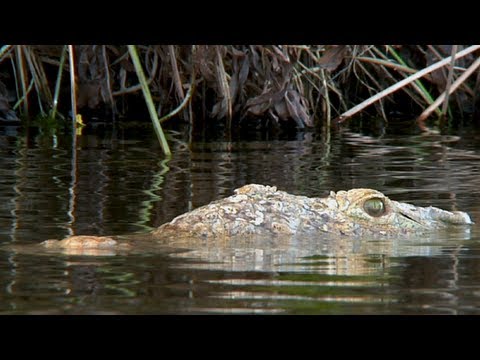This outdoor photo captures a serene swamp scene framed by thick black borders on the top and bottom. The background features tall grasses and weeds in varying shades of green, gray, and brown. Calm waters with visible ripples dominate the middle of the photo, reflecting the surrounding vegetation. Central to the image, an alligator floats partially submerged, its body extending from the left to the right. Its closed mouth straddles the waterline, with a prominent, dark brown eye that appears to be staring outward. The alligator's textured scaly skin showcases a combination of light brown, medium brown, and grayish-tan hues, with a small hump on its back leading into its tail. The overall atmosphere of the photo suggests a tranquil yet watchful moment in the swamp.